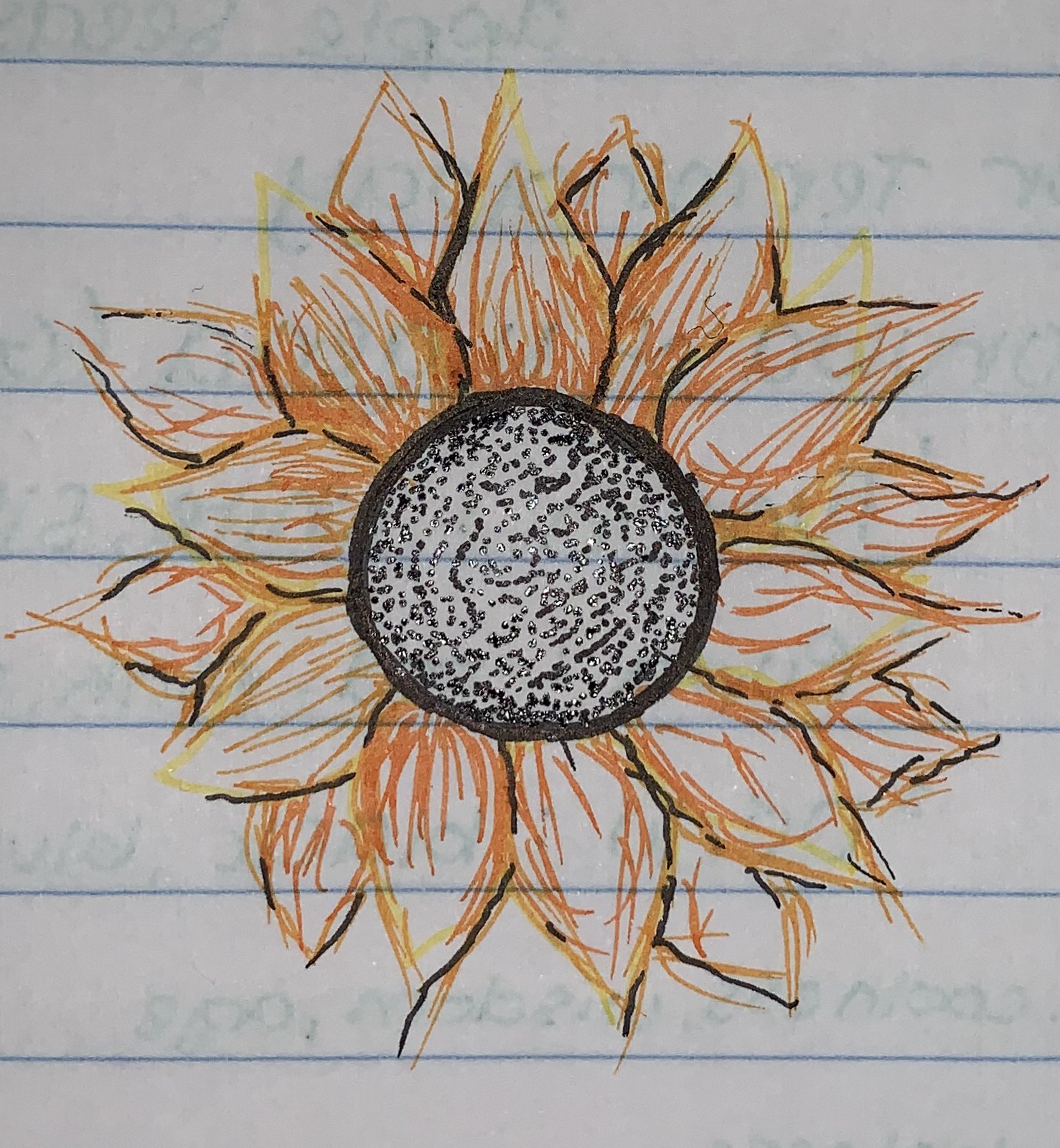The image depicts a large, intricately detailed drawing of a sunflower, likely created by a child using felt-tip pens on a piece of white writing paper with widely spaced blue lines. The sunflower, dominating the entire sheet, features a prominent black circle in its center filled with black and silver speckles, evoking the texture of sunflower seeds. Radiating from this center are two interleaved rings of petals, marked with faint black outlines. The inner ring contains nine orange petals with distinctive streaks, while the outer ring displays additional petals with tips colored in orange and a little yellow, giving a fiery, dynamic feel as if the petals are in motion. Notably, the drawing lacks a stem, focusing solely on the vibrant flower head. The reverse side of the paper contains some indistinct writing, partially visible through the drawing.